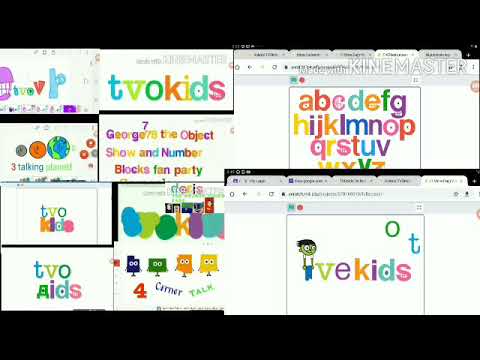The image features a black border at the top and bottom, with two web browser windows displayed on the right side. Both browser windows have five tabs open at the top. The upper browser window shows a box containing the alphabet, though the letters "W," "X," "Y," and "Z" are cropped out at the bottom. This is because the lower browser window is superimposed on top of the upper one.

In the lower browser window, there is a box displaying a cartoon caricature of a person. Beside this caricature, the letters "V E K I D S" are visible. Above this box are the letters "O T," and to the left of it, there are several smaller white boxes. One of these smaller boxes contains an image of the Earth with text that is too small to read. Another box is labeled "Georgia's The Object Show and Numberblocks Fan Party." Below these boxes, there appear to be images resembling four different states.